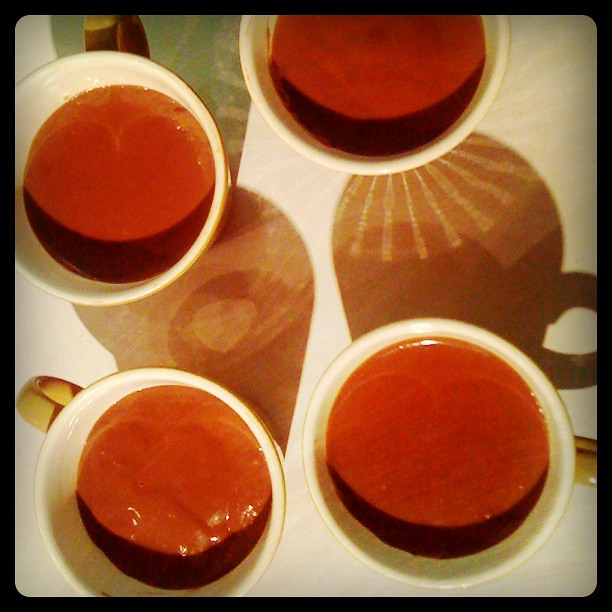This image showcases a top-down view of four medium-sized white coffee cups with off-yellow handles, arrayed on a light wooden table. The cups cast overlapping shadows on the table, indicative of a lighting source directly above. Inside each cup is a thick liquid with a reddish-brown hue, suggesting it could be a rich tomato soup or possibly a pudding, rather than coffee due to its dense appearance. The consolidation of light and the shadows creates an interesting visual effect, enhancing the color and texture of the substance inside the cups.